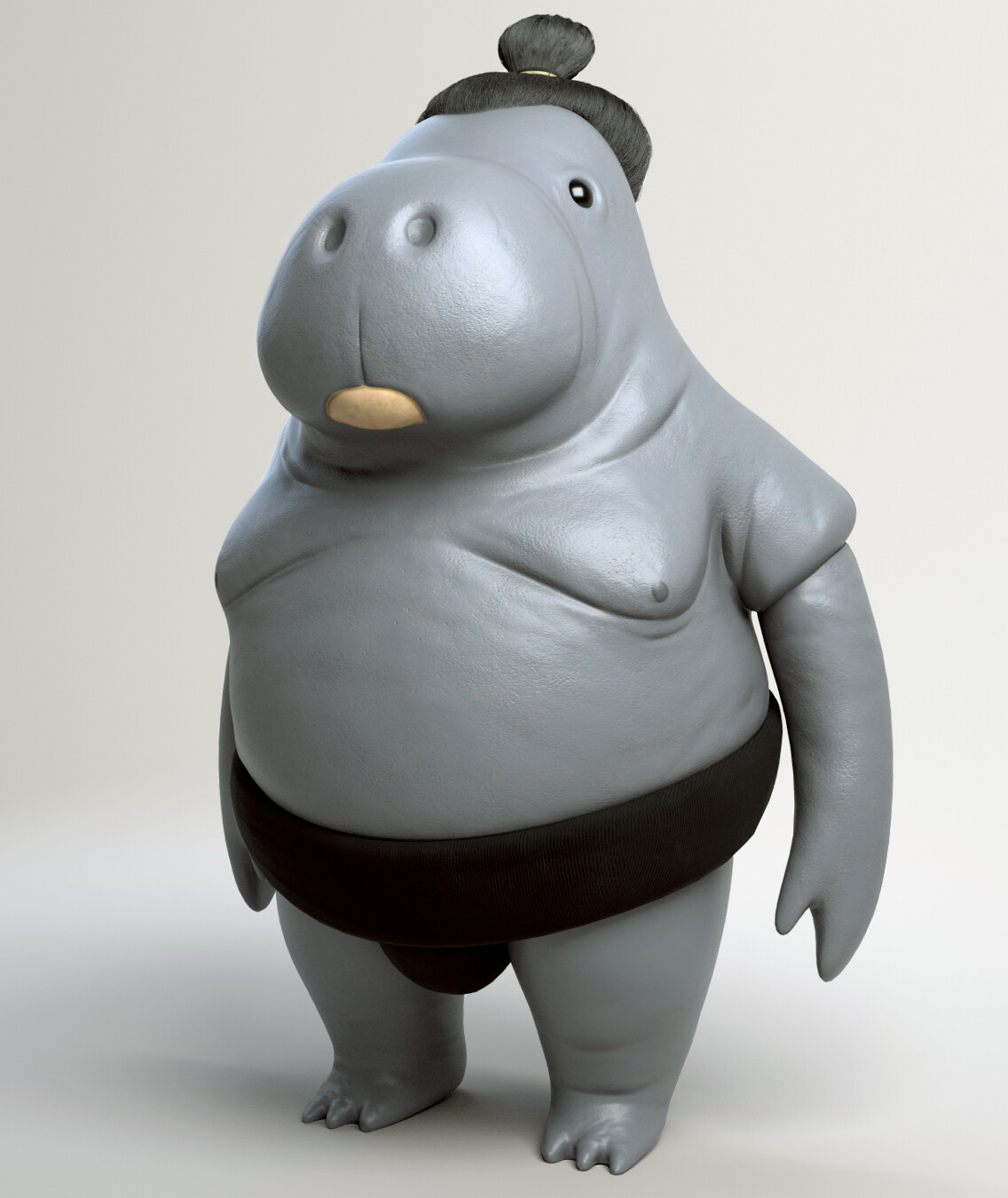This detailed sculpture portrays a whimsical fusion of a hippopotamus and a sumo wrestler, standing upright like a human. Crafted from a gray material, likely clay, it features the unmistakable large snout and eyes characteristic of a hippopotamus. The eyes are black, with one facing the camera. Adding to its sumo wrestler likeness, the sculpture's black hair is styled into a traditional sumo wrestler's bun or ponytail.

The figure's physique is notably rotund, with a prominent belly and exposed chest displaying sagging breasts, suggesting an exaggerated sense of mass and volume typical of sumo wrestlers. It wears the dark mawashi, the distinctive bottoms worn by sumo wrestlers, offering a humorous contrast to its otherwise animalistic form. Its thick, bare legs end in flat feet with three toes each, firmly planted on the ground. The arms are more stylized than realistic, exhibiting extra flesh on the upper parts. The mouth is slightly open with the tongue playfully sticking out, contributing to the overall humorous and contemporary feel of the sculpture.